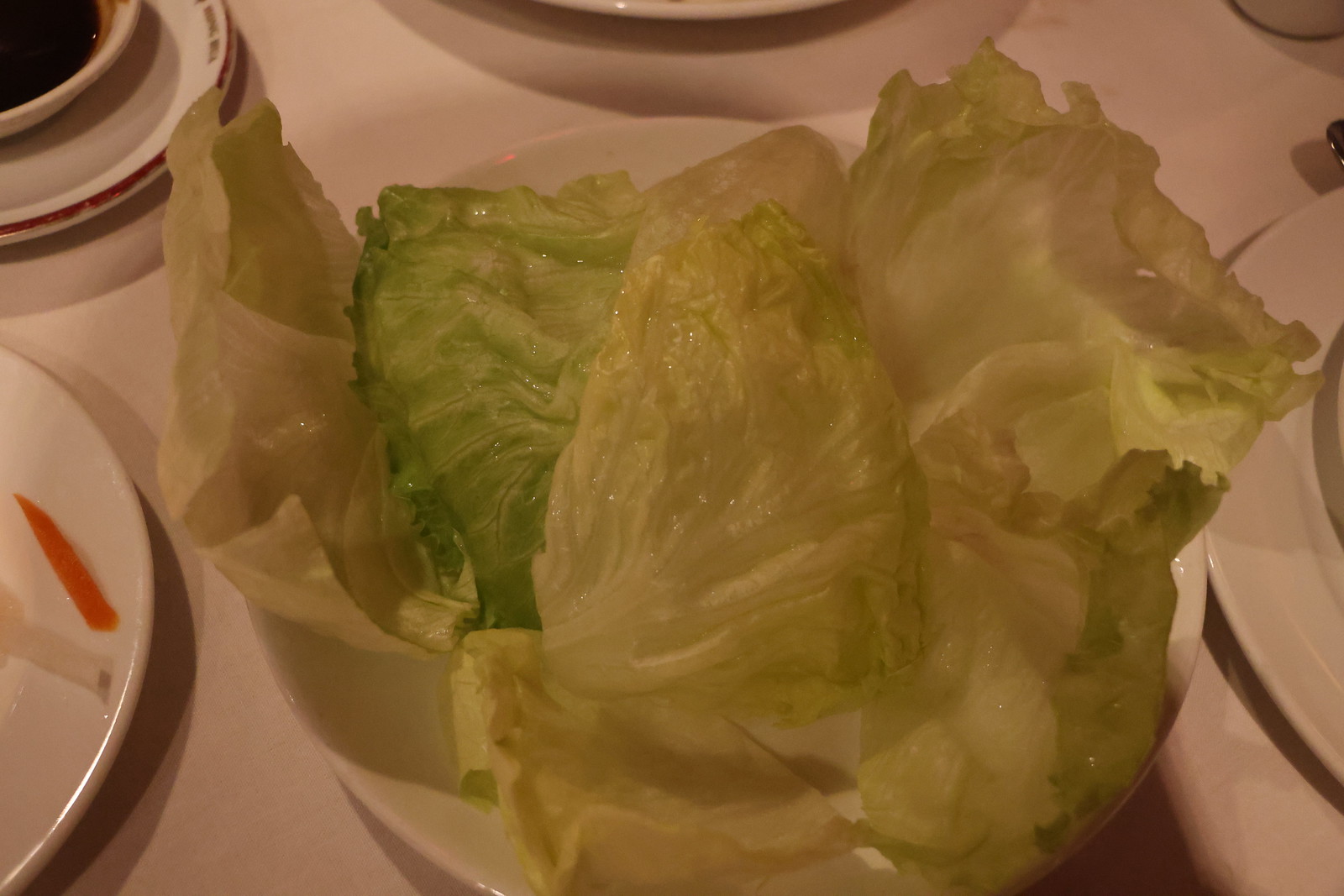This close-up image captures a meticulously arranged table setting on a white tablecloth. Dominating the center of the composition is a white plate holding vividly crisp iceberg lettuce leaves, predominantly yellowish-green with hints of darker green towards the base, arranged such that several stand upright, lending an organic texture. Positioned to the lower left is a larger white plate with a distinct piece of red or orange, possibly a carrot or pepper, adding a pop of color. The upper left corner features a stack of two white bread plates, above which is a white saucer with a dark liquid, suggestive of coffee or sauce. Toward the top center, the edge of another large plate can be seen, hinting at a layered presentation. In the upper right, part of another bowl emerges into view, with what seems like a utensil resting on a nearby white dish. Overall, the image meticulously details a sophisticated, monochrome dining arrangement punctuated by strategic splashes of color from the vegetables.